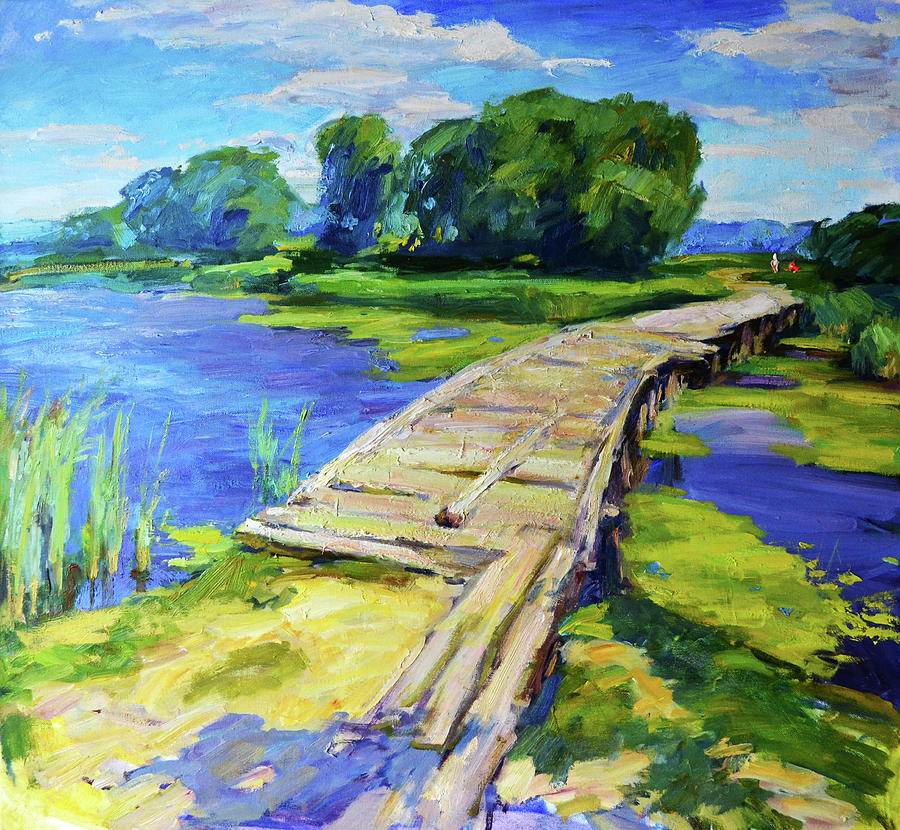This is a square oil painting characterized by visibly thick and intentional brush strokes. At the center of this image lies a serene river, flowing from right to left at a slight diagonal with vibrant blue water that extends into the distance. A rustic wooden footbridge, constructed from light brown logs and wooden planks, spans the river, connecting its shores. The water's surface in the foreground is interspersed with patches of green algae or moss, while tall reeds grow along the river's edge on the left side.

The scene on the far shore of the river features a lush green expanse of grass dotted with several green trees. Beyond the bridge, a small dirt path bordered by more trees stretches into the distance. Notably, two bright red figures, likely people, are visible in the background, adding a focal point to the tranquil setting. The sky is painted in soft hues of blue, with white and slightly gray clouds scattered across it. The subtle texture of the canvas adds depth to this detailed and highly textured landscape.